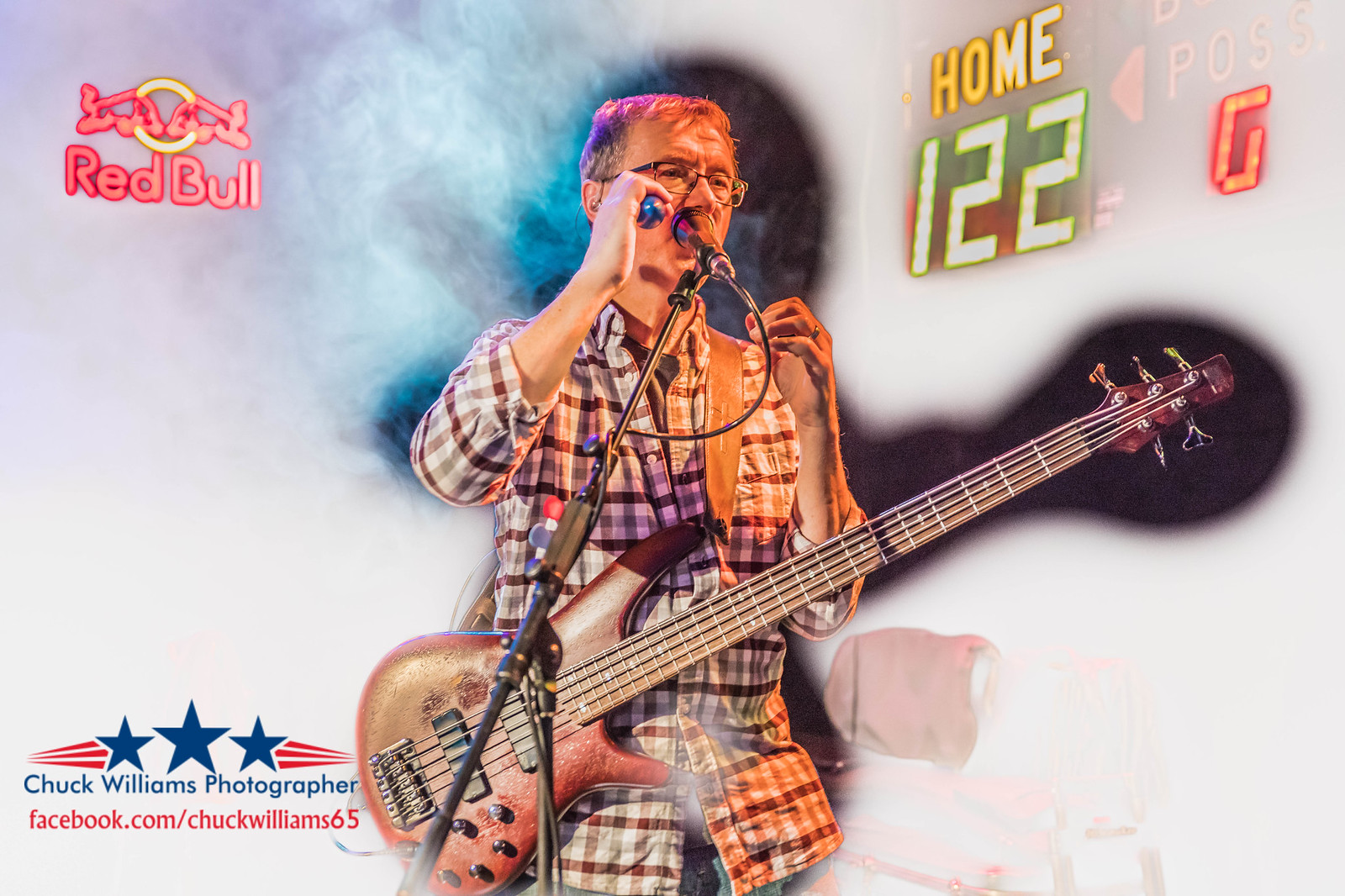The image depicts a musician on stage holding a five-string bass guitar with a brown finish. He is wearing a checkerboard-pattern flannel shirt and glasses, and is positioned in front of a microphone, appearing to speak into it. In his right hand, he holds a spherical object while a guitar strap hangs around his shoulders. The background features a neon Red Bull logo on the top left and a basketball-style scoreboard reading "HOME 122," with possession markers and a zero. The bottom left corner includes the text "Chuck Williams Photographer" along with a logo adorned with red and white stars and stripes, as well as a Facebook link to "facebook.com/ChuckWilliams65." The scene is enveloped in thick, foggy smoke, which appears to have been edited using Photoshop to make the musician more visible. The overall impression suggests a promotional effort by the photographer, Chuck Williams, using a creatively altered stage performance image.